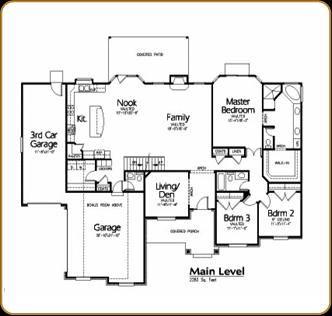This image showcases a detailed floor layout blueprint of a residential property, likely a house or apartment. The blueprint is set against a black background with a central white square containing the floor plan.

Starting from the left side, the layout features a tall vertical rectangle labeled "Third Car Garage." Adjacent to this is a large room divided into two sections: the left side marked as "Nook" and the right side labeled "Family." Below this, there is another square labeled "Garage," situated underneath the "Nook." A room labeled "Living/Den" is positioned between the garage and the family room.

To the right of the "Living/Den" is a smaller, somewhat difficult to decipher room. Additionally, next to this smaller room, there is a rectangular room labeled "Bedroom 3." Heading further right, another square room marked "Bedroom 2" is adjacent to Bedroom 3. 

Above Bedroom 2, there is a square room connected to what appears to be a bathroom. To the left of this bathroom and above the family room, the layout indicates the "Master Bedroom," which is connected to the family room and the nook. Adjacent to this area, at the top, is another distinct square room with illegible writing.

At the bottom of the blueprint, the words "MAIN LEVEL" are prominently displayed in bold black letters. Below this, smaller text likely includes details such as an address, price, or the total size of the property, though it is not clearly legible in the image.